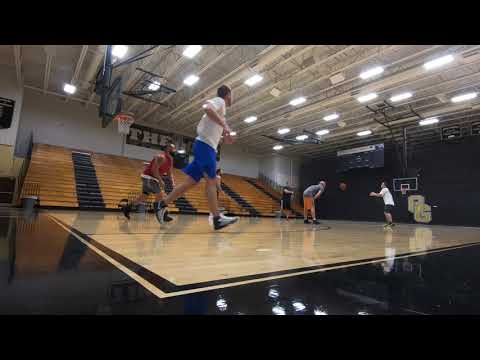This photograph captures an indoor basketball game in a gymnasium. The image is taken from ground level with a wide-angle lens, emphasizing the shiny light wooden court, outlined in black. Both basketball hoops are visible, and the bleachers are extended but empty. The gym is brightly lit with fluorescent lights and no natural light. In the game, which looks like a small pickup match of two-on-two or three-on-three, players are dynamically positioned. One player in blue shorts and a white shirt is nearest to the camera, while another in orange shorts and a gray shirt is further away. A player in brown is passing the ball to someone in a white t-shirt. The ball can be seen in mid-air moving towards the far hoop. A black banner with the partially visible word "THE" hangs on the upper part of a white wall at the far end. The scene exudes an atmosphere of casual yet energetic practice or friendly scrimmage without any audience or scoreboard present.